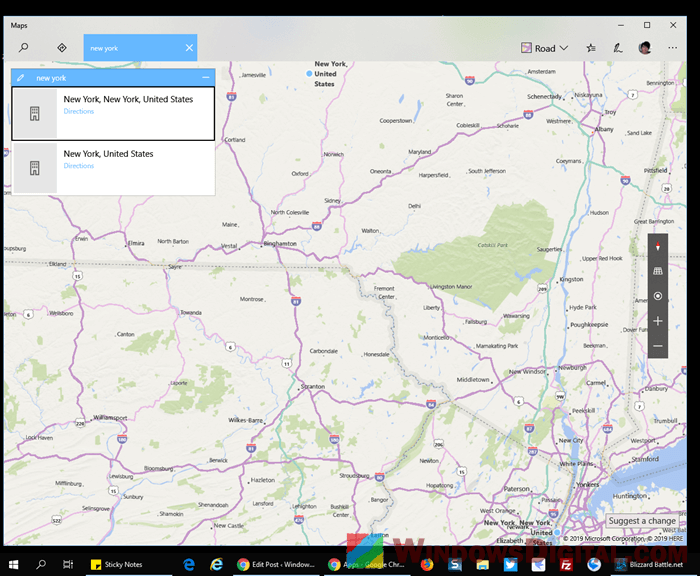Screenshot of a digital map interface displayed within a Windows operating system window. The familiar Windows taskbar is visible at the bottom of the screen. The application’s interface includes a gray title bar at the top, with "Maps" displayed in the top-left corner and the typical Minimize, Maximize, and Close buttons in the top-right corner.

Beneath the title bar, there is a navigation section. On the left, a search icon resembling a road sign is visible. Adjacent to it, there is a blue tab labeled "New York" in white text, accompanied by a white "X" on the right side of the tab. To the right of the blue tab, there is a drop-down menu labeled "Road," followed by several icons: a star, a pin, a user profile picture, and the three horizontal dots representing additional options.

The main portion of the window is occupied by the map. On the map, "New York, New York" is indicated towards the bottom-right corner, while "New York, United States" is marked at the top with a prominent blue circular pin. The map’s roads are illustrated in purple, providing a distinctive visual detail.